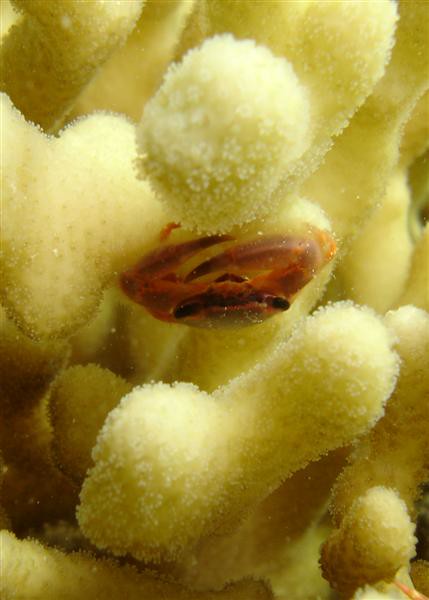This underwater photograph captures a detailed and vibrant scene from the ocean floor or possibly an aquarium setting. Dominating the image are yellow, bulbous sea sponges, appearing soft and squishy, almost furry in texture. Tiny bubbles float around, adding to the aquatic ambiance. In the center of the image, a small red crab with prominent black eyes and distinct left and right pincers takes the spotlight, nestled between the sea sponges. Its vivid red color contrasts beautifully with the amber and gold hues of the surrounding environment. Additionally, a small brown fish can be seen swimming amongst the sponges, adding life and movement to the serene underwater tableau.